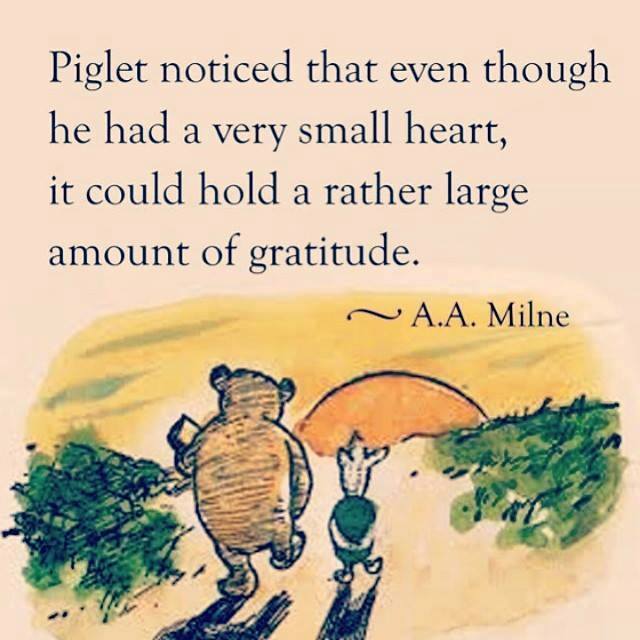The image features a heartwarming scene set against a pale pink background, combining a poignant quote with a charming illustration. At the top, blue text reads:

"Piglet noticed that even though he had a very small heart, it could hold a rather large amount of gratitude."

Beneath the quote, the illustration depicts Winnie the Pooh and Piglet walking side by side across a gently sloping grassy field. Pooh, who is on the left, carries what appears to be a jar of honey in his left hand, while Piglet is on the right with his arms clasped behind his back. The scene takes place under a golden sky that suggests the sun is setting, casting a warm glow over the landscape. There are patches of shrubbery on the left and more grass on the right, adding to the idyllic feel of the scene. Below the illustration, the text "A.A. Milne" credits the quote to its author. Overall, the image evokes a sense of gratitude and friendship, beautifully captured in a watercolor-like style.